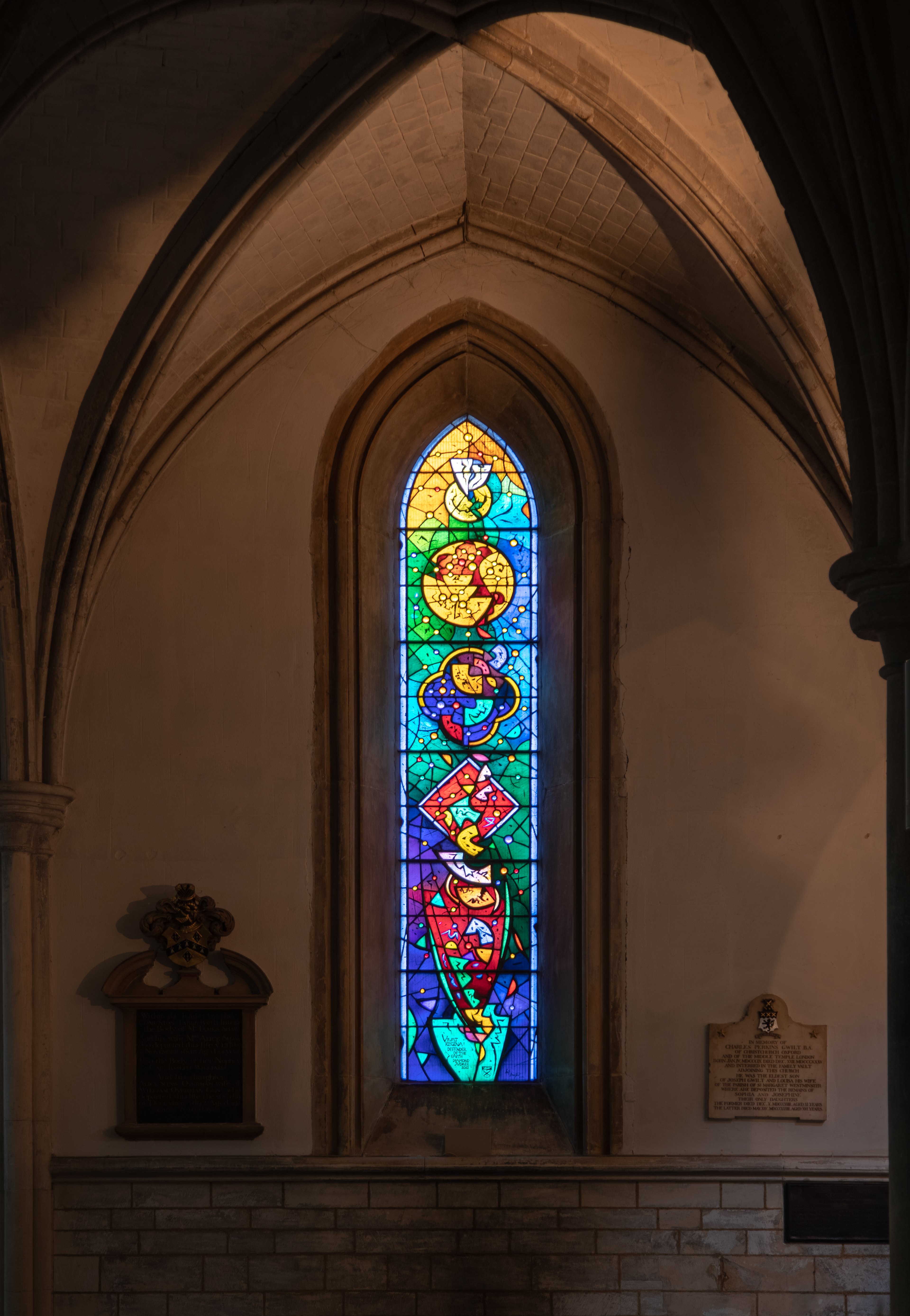The photograph captures the interior of a dimly lit church, specifically focusing on a towering stained glass window. The window, set within a smooth stone frame that curves inwards, features a pointed arch at the top, reminiscent of medieval church architecture. The wall beneath the window transitions from brick at the base to a smoother, white surface, flanked by two plaques that remain largely illegible due to the darkness.

The stained glass itself is a vibrant mosaic of colors and shapes, composed of six distinct sections. At the very top, a small sphere with an object resembling a dove sits amidst a predominantly yellow and green palette. Below this, a yellow circle with an orange core is followed by a dark blue, rounded four-sided shape. The fourth section features a diamond shape with reds and yellows, and the fifth consists of a distinct red triangular design. The final section at the bottom portrays a light blue triangular shape, potentially resembling a shield.

Despite its abstract nature, the stained glass window is the focal point of the image, with light filtering through its vivid colors, casting intricate patterns inside the church. The vaulted ceiling and surrounding details add to the reverent and historical ambiance of the scene.